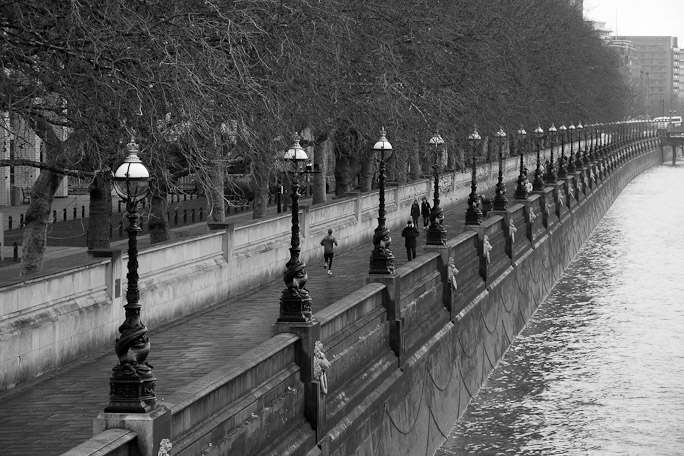In this detailed black-and-white photograph, we observe a tranquil river walk scene. On the right side of the image, a calm body of water edges against a raised, concrete embankment. Adjacent to this body of water, moving leftward, is a sidewalk reminiscent of a bridge or walkway, adorned with evenly spaced lampposts approximately every 10 to 20 feet. The lampposts line the pathway, gently curving into the distance. The scene is bustling with activity as various people stroll and jog along the riverside promenade. Trees, devoid of leaves, suggest a winter setting and contribute to the monochromatic palette of black, white, and gray shades that dominate the photograph. In the backdrop, buildings, both near and far, populate the skyline, hinting at a downtown or park-proximate location. The overall arrangement of objects appears scattered yet harmonious, encapsulating a blend of nature and urban life. The photograph is marked by a watermark in the bottom right corner, "Tim Jackson Photography," discreetly inscribed in the otherwise detailed and immersive composition.